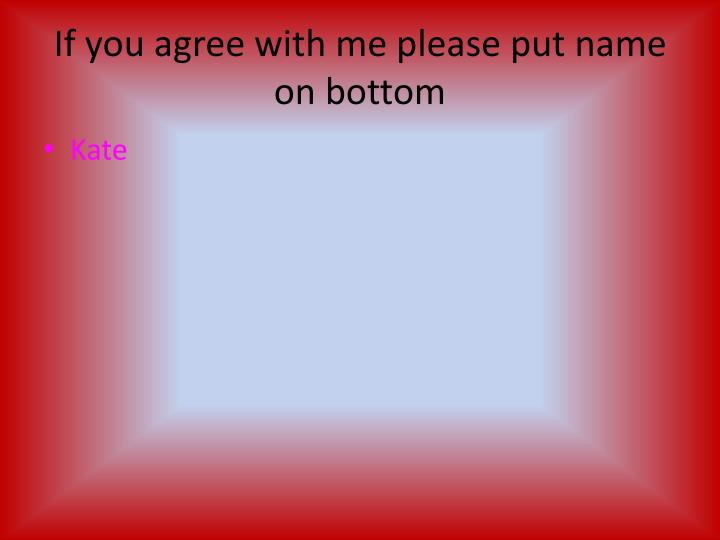The image depicts a squarish, PowerPoint template-like graphic with a red border that transitions into a gradient of white in the center, creating a starburst effect from white to light pink to red. At the top of the image, in a simple black font, are two lines of text stating, "If you agree with me, please put name on bottom." Below this, to the left, is a single bullet point in pink text that reads "Kate." The overall background features a gradient radiating from a central rectangular "window" of brightness, blending red into white and light pink as it extends outwards, giving the appearance of light radiating into a reddish-pinkish backdrop. The image likely represents a petition or the conclusion of one, indicating a request for signatures with one name already appearing.